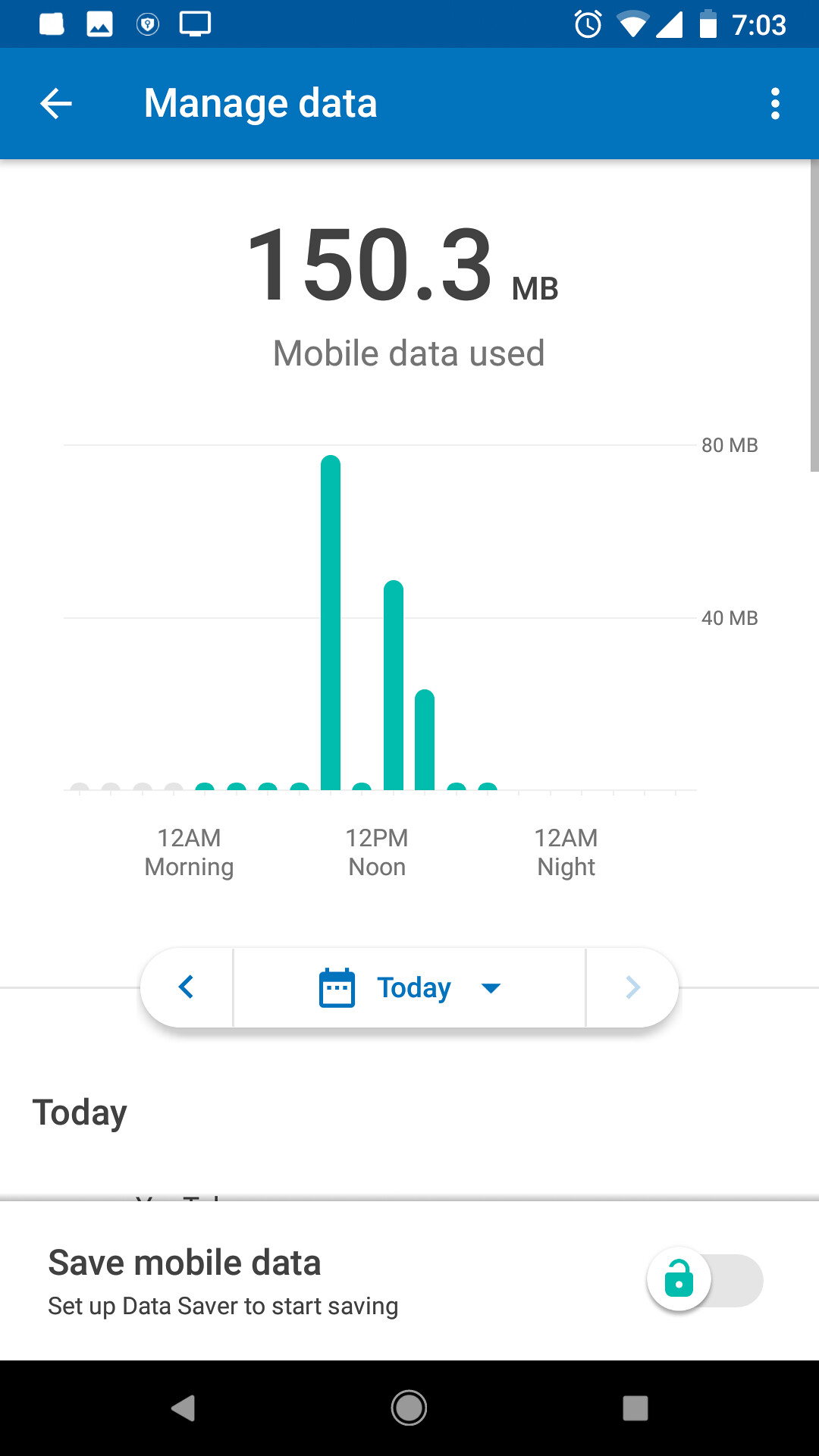This image is a detailed screenshot of a phone's settings menu, specifically displaying the user's mobile data usage. The header, "Manage Data," is highlighted in a sky blue color at the top of the screen. Below it, the current data usage is indicated as 150.3 MB. 

A detailed graph below the data usage summary visually represents mobile data consumption over a 24-hour period, with time stamps at 12 a.m. (midnight), 12 p.m. (noon), and 12 a.m. (midnight). The graph features bars illustrating the data used at specific times, showing peak usage around noon, with the values spiking probably between 40 MB and 80 MB.

Further down the screen, there is a feature to select specific dates to review data usage history. Beneath this section, a text prompt reads, "Save mobile data, set up Data Saver to start saving," accompanied by a sliding button icon, which likely toggles the Data Saver feature on or off.

The bottom portion of the screenshot shows the default black bottom bar typical of Android phones, including the home screen navigation buttons. 

At the top of the screen, it's displayed that the time is 7:03, the phone has a three-quarters battery charge, is connected to Wi-Fi, and has cellular service. Additionally, there's an alarm icon, suggesting an alarm is set. There are four other unidentified icons on the left-hand side of the status bar.